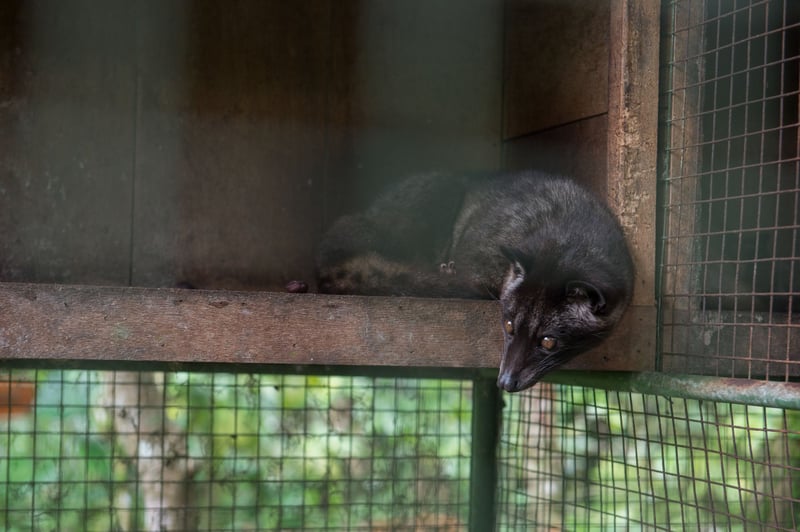The image depicts a small, black-furred creature with brown eyes resembling a combination of a cat and a fox, sitting atop a tipped wooden box. The animal has a pointed nose and a coat speckled with hints of white. It appears to be lying in the box with its head hanging over the edge, seemingly watching something to its left and looking somewhat threatened. Surrounding the wooden box are sections of a green, grid-like cage, indicating it might be enclosed within a larger caged environment, reminiscent of zoo enclosures. To the right of the box, there's a similar grid-like structure, but this one is rusted, adding a rustic touch. In the background, there's foliage visible through the mesh screens.